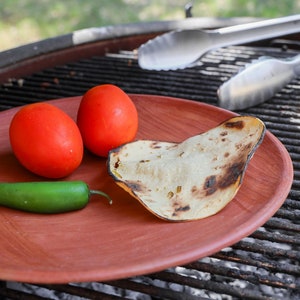The image is a food advertisement or food article close-up of a salmon-colored, clay-styled, circular plate set on an outdoor grill. The grill bars appear covered in gray ashes and charcoal, indicating it's not in use. On the plate, there's a slightly burned, small flatbread, possibly a tortilla. Positioned to the upper left of the tortilla are two round, red fruits, resembling tomatoes or potentially hard-boiled eggs. Below these and to the left of the tortilla lies a slender green chili pepper. A pair of metallic, silver-toned tongs with only the head clippers visible are placed in the background, adding context to the grilling scene. Blurred greenery in the upper background further suggests an outdoor setting.